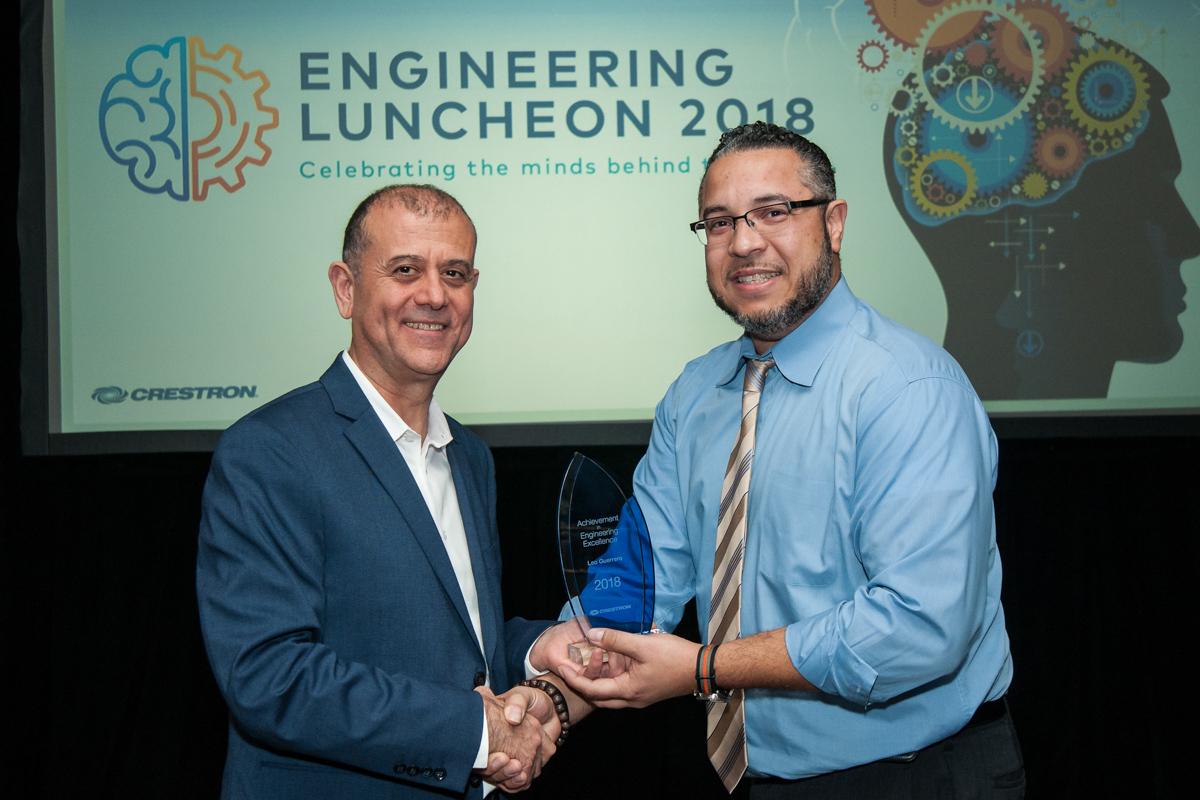In this image, two men are standing on a stage, shaking hands and holding a clear glass trophy with partial text that includes the year 2018. The man on the right is dressed in a blue long-sleeve shirt with a tie featuring diagonal stripes in white, yellow, and brown, and he wears glasses. The man on the left is wearing a white shirt under a blue suit jacket. Behind them, a large screen displays text at the top that reads "ENGINEERING LUNCHEON 2018" in blue, followed by "Celebrating the minds behind" in green. The last word is obscured. On the screen's right side, there’s an image of a head silhouette with an engine or gears inside it, stylized in multiple colors, embodying a fusion of a brain and mechanical elements. The screen features a logo or sponsorship from a company, possibly Crestron.